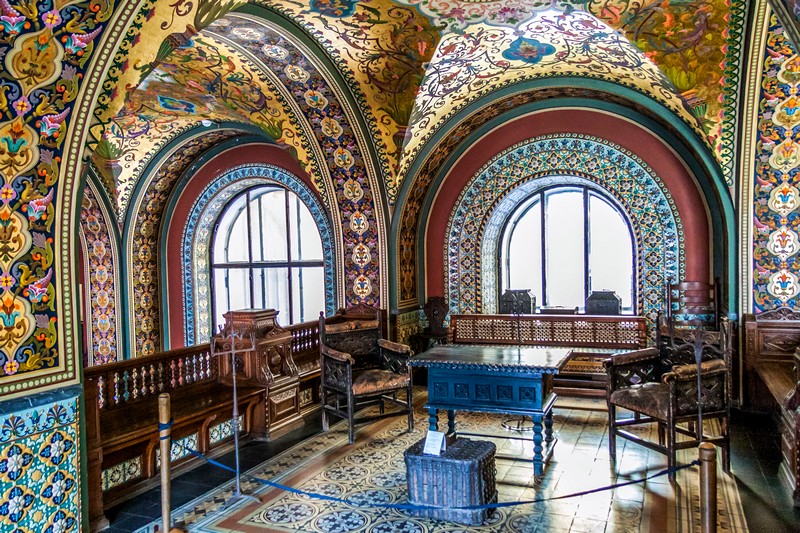This highly detailed, full-color indoor photograph captures an opulent and vividly ornate room, suggestive of religious or historical significance possibly within a museum setting. The square image, devoid of a border, immerses the viewer in a room practically bursting with color. Dominated by extravagant decorations, the walls and floor showcase intricate designs in vivid hues, including an abundance of yellows, browns, and greens, which give a sense of the richness and historical value encapsulated in this space.

Central to the image are two oval-shaped windows with protective bars, framed by elaborate decorations comprising eight concentric ovals that amplify the room's grandeur. Adding to the ornate ambiance, what appears to be tapestries or carpets drape the walls, elevating the luxurious appeal. Furniture pieces, including a prominently situated wooden table and chairs, emphasize the room's functionality while blending seamlessly into the ornate surroundings. A roped-off area and a box with an attached placard perhaps indicating an exhibit or an important artifact, underscore the potential museum context, suggesting that significant investment has gone into preserving this visually captivating, historically treasured room.